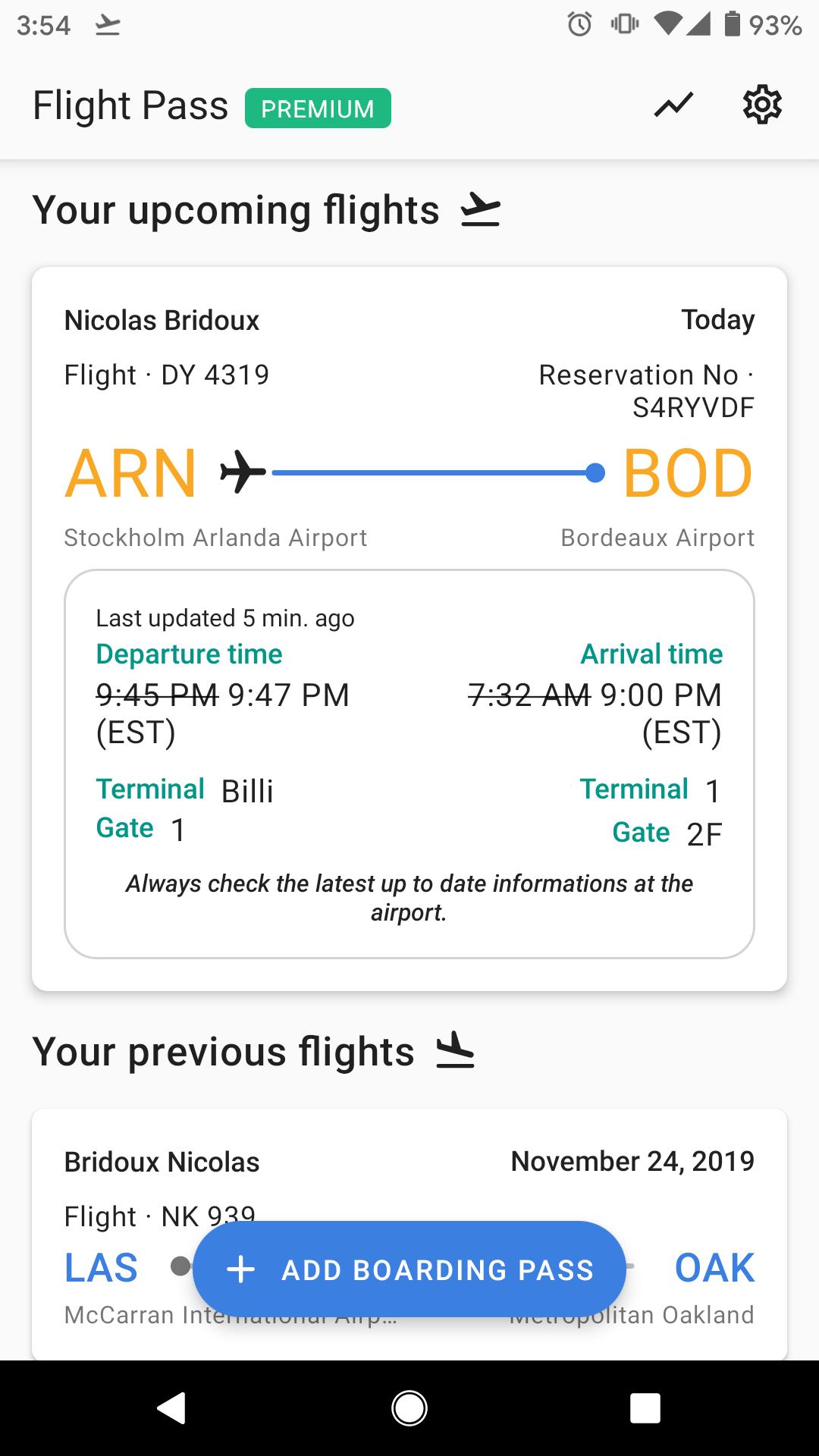**Detailed Caption:**

The on-screen image captures a mobile device's display, showcasing several status icons at the very top, including the time at 3:54, airplane mode, alarm clock, vibrate, Wi-Fi, and a battery icon indicating a 93% charge. Below these icons, a green banner labeled "Premium" is prominently displayed, nestled within a section titled "Flight Pass," accompanied by a settings icon on the far right.

Further down, the screen presents information on upcoming flights, with a black silhouette of an airplane and a depiction of a travel ticket. The ticket features the name "Nicholas Bridox" and provides details for flight DY 4319, which is scheduled to depart from Stockholm Orlando Airport to Bordach's Airport. The accompanying reservation number is S4RYVDF.

A highlighted box beneath this information states it was last updated five minutes ago. The revised departure time is noted as 9:47 PM Eastern Time, departing from Terminal Billy, gate 1. Additionally, the expected arrival time is marked at 9:00 PM at terminal 1, gate 2.